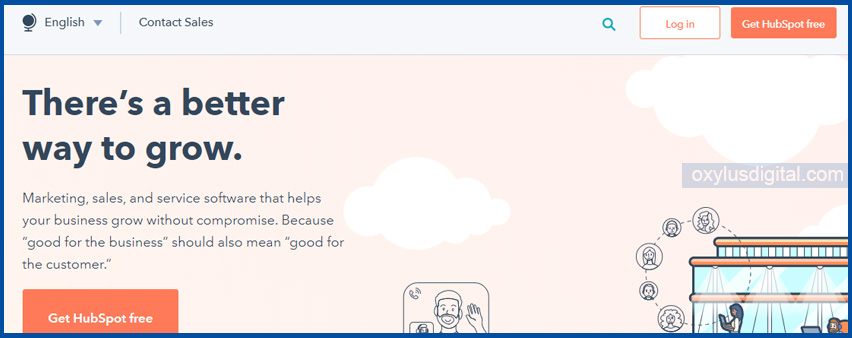This image is a screenshot from an unspecified source, primarily focused on promoting HubSpot. At the top of the screenshot, a navigation bar displays options such as "English," "Contact Sales," "Search," "Log in," and "Get HubSpot free." The main text highlights a marketing message: "There's a better way to grow. Marketing, sales, and service software that helps your business grow without compromise. Because good for the business should also mean good for the customer. Get HubSpot free."

The visual elements include a cartoon illustration of a man on a FaceTime call, waving at the camera. In the bottom right corner, there's an image depicting a building where people inside are working on laptops. This section is marked with a watermark reading "OXYLUSdigital.com." The entire image is encased in a blue border. Notably, the image is taller than it is wide and contains no photographic elements or real-life subjects, such as people, animals, plants, or landscapes.